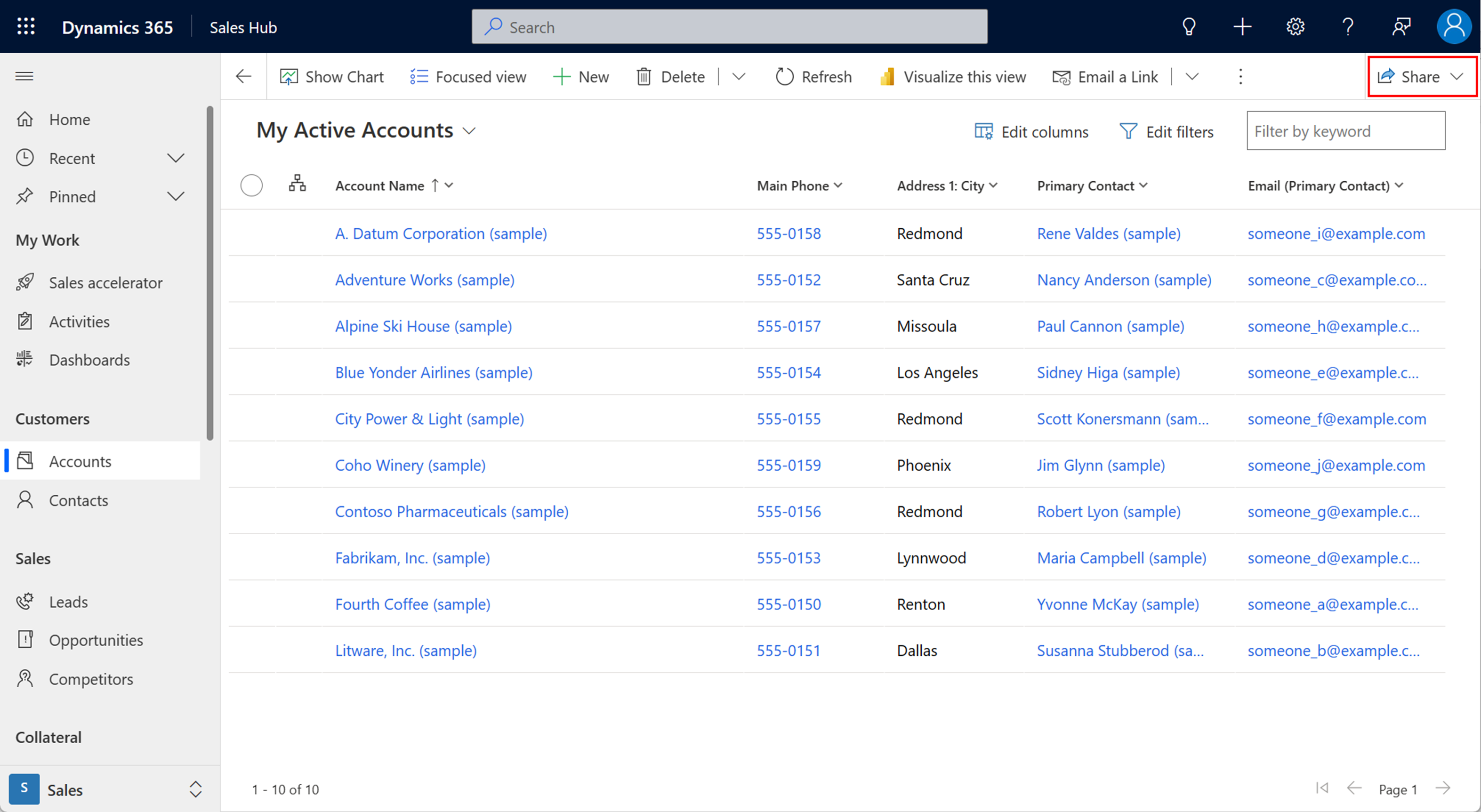The image is a screenshot of the Dynamics 365 Sales Hub web page. At the top of the page, there is a black navigation bar displaying the title "Dynamics 365 Sales Hub". To the right of the title, there are several icons: a search bar with a magnifying glass, a light bulb, a plus sign, a settings gear, a question mark, a people icon, and a blue circle with a person icon inside it.

On the left side of the page, a vertical menu lists the following options: Home, Recent, Pinned, Sales Accelerator, Activities, Dashboards, Accounts, Contacts, Leads, Opportunities, Competitors, Collateral, and Sales.

Directly below the main black navigation bar, there is another toolbar with options labeled: Show Chart, Focused View, New, Delete, Refresh, Visualize This View, Email, Link, and Share.

The primary section of the page is titled "My Active Accounts" in bold, followed by options to Edit Columns, Edit Filters, and Filter by Keyword. Below these options, the account list is displayed with the following column headers: Account Name, Main Phone, Address, City, Primary Contact, and Email.

The account list itself is shown in blue and includes the following entries, each with associated details such as phone numbers, addresses, contacts, and emails:
1. Adatum Corporation | Phone: Sample 5550158 | Contact: Rene Valdez | Email: someone@example.com
2. Adventure Works
3. Alpine Ski House
4. Blue Yonder
5. City Power and Light
6. Coho Winery
7. Contoso Pharmaceuticals
8. Fabrikam Inc.
9. Fourth Coffee
10. Litware

Each account name is listed alongside its respective phone number, address, contact person, and email address, organized in a vertical sequence.